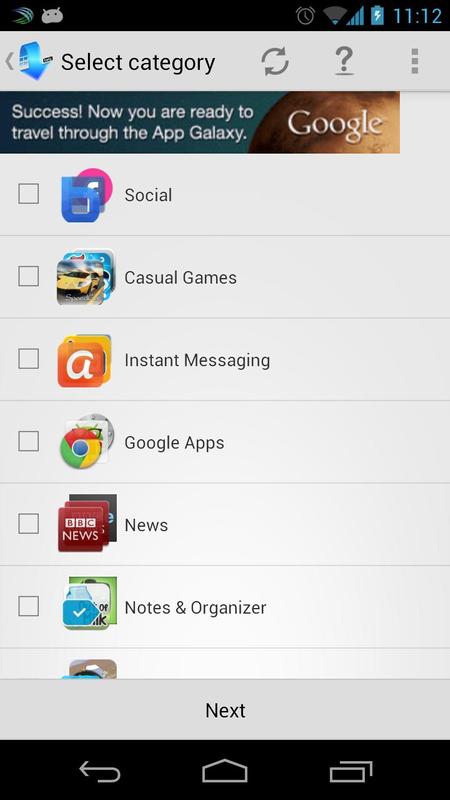The screenshot captures a phone interface. In the upper right-hand corner, there is a timestamp of "11:12," along with an icon indicating full battery life with the device currently charging. At the top of the screen, the title "Select Category" is prominently displayed. Below this, a message within a bar reads, "Success. Now you are ready to travel through the App Galaxy," accompanied by the Google logo on the right.

The main section of the screen comprises several rows. Each row contains an empty checkbox on the left, followed by a logo, and then some black text describing the category. The categories listed are:

1. Social
2. Casual Games
3. Instant Messaging
4. Google Apps
5. News
6. Notes and Organizer

Below these rows, a light gray band spans the width of the screen, featuring the word "Next" in black text at its center. Further down, a black navigation bar includes three icons: a curved arrow pointing left on the right, a minimalist house shape in the center, and a narrow rectangle with two lines above it on the top and right side on the left.